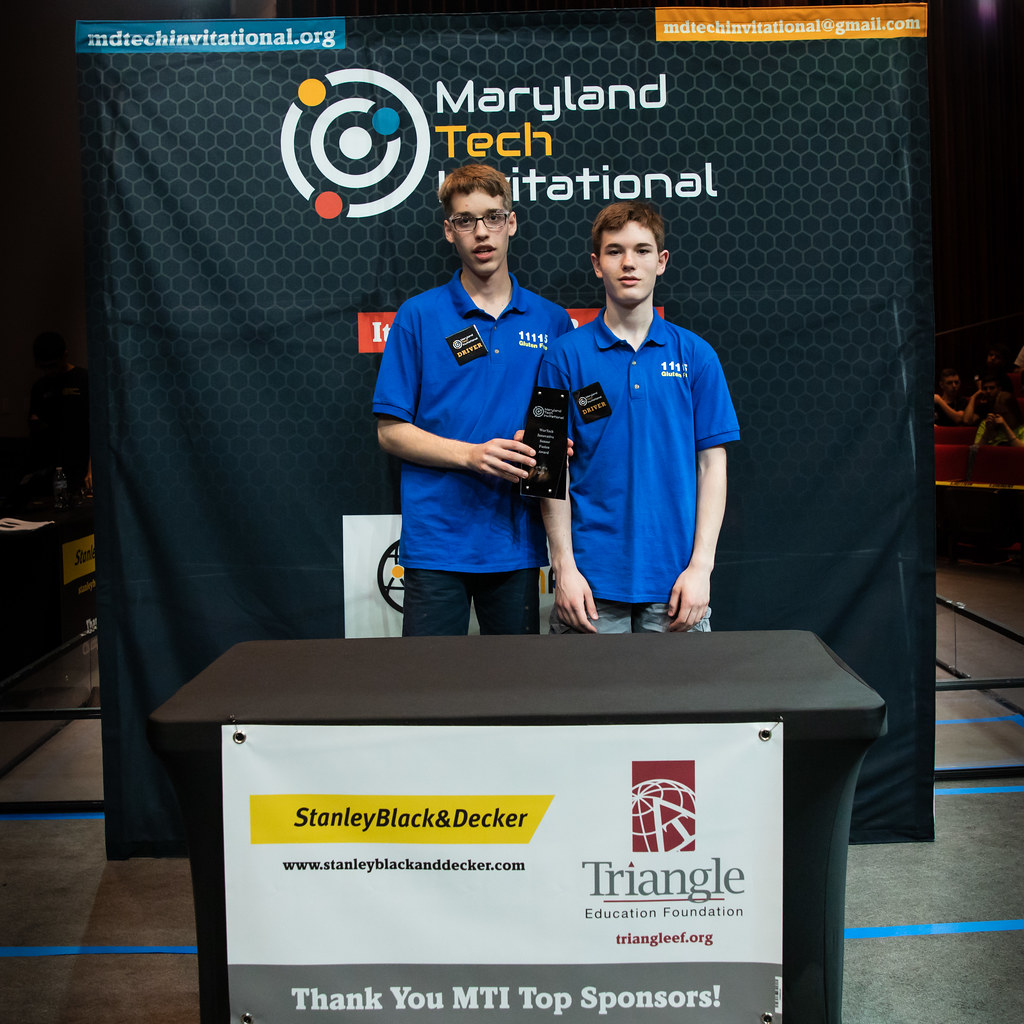The photograph features two young boys, likely in their early teens, standing in front of a visually detailed backdrop and podium at an event. The backdrop is a black banner that reads “Maryland Tech Invitational” along with its web address, "MDTechInvitational.org," and its email, "mdtechinvitational@gmail.com." The banner is emblazoned with concentric circles in white, yellow, red, and blue, and highlights the word "Tech" in yellow with "Maryland Invitational" in white.

Both boys are dressed in ocean-blue short-sleeve T-shirts. The boy on the left wears black pants, while the boy on the right has on light blue jeans. Each boy sports a black tag with the word "driver" on it, and part of a number "11115" on the left boy's shirt is visible. They are positioned in front of a black podium that has a sign promoting “Stanley Black and Decker” with its website "www.stanleyblackanddecker.com" printed in black on a yellow background.

In addition to the main banner, there's another sign on the right with the logo and name of the Triangle Education Foundation, featuring text in gray and burgundy. The setting has a combination of gray and black flooring with white lines, providing a modern industrial atmosphere to the tech-related event.